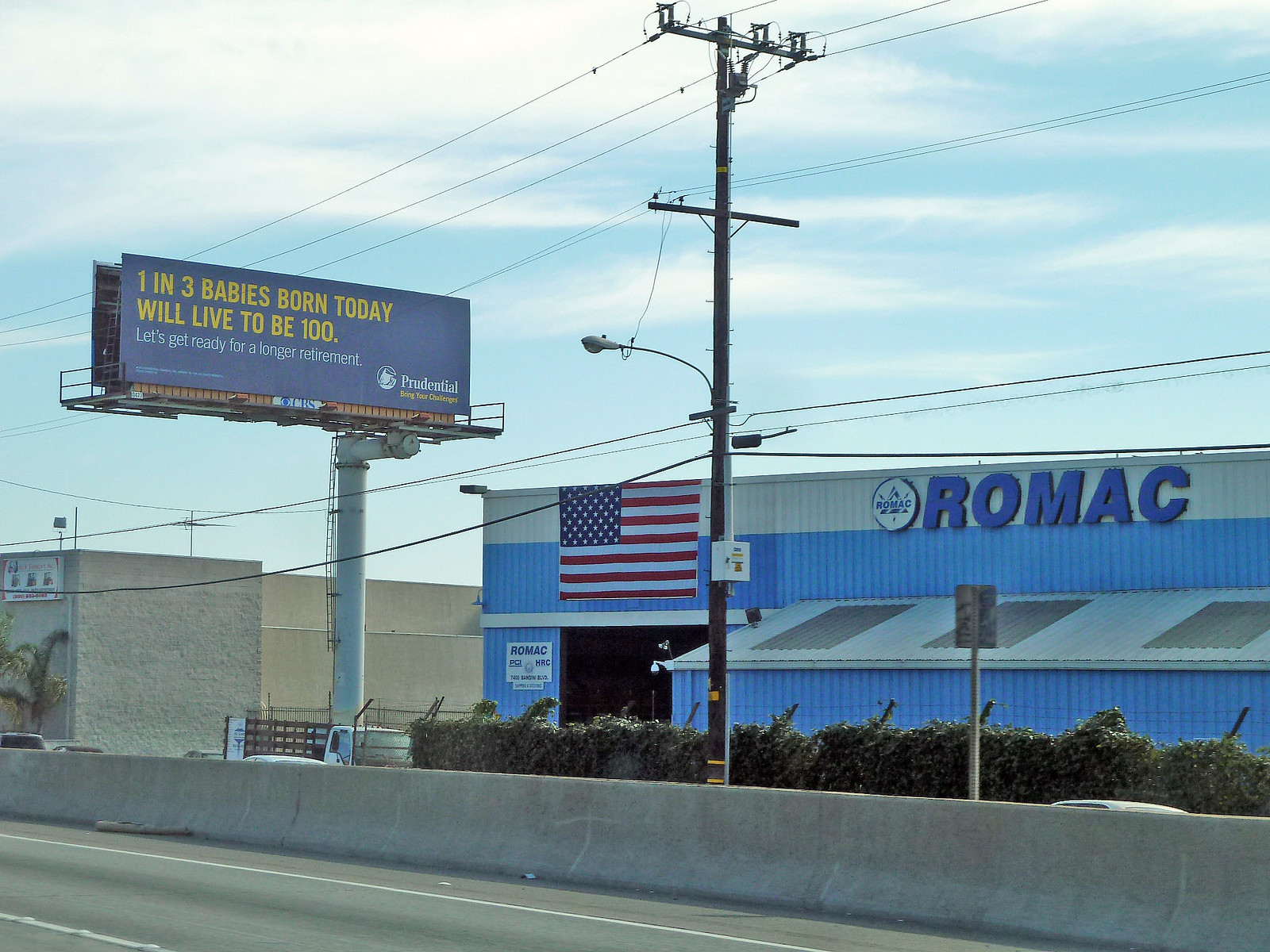A rectangular photograph captures a scene from a freeway, with the longer side of the rectangle stretching horizontally. Dominating the image is a central telephone pole that emerges prominently from the barrier dividing the freeway from the adjacent road. This pole extends nearly to the top edge of the photo, and features multiple wires branching out at different points, as well as a street light about halfway up.

To the left of the telephone pole, a billboard rises, supported by a single pole. The billboard has a blue background with striking yellow and white text. The yellow text reads, "One in three babies born today will live to be 100." Below that, in white text, it reads, "Let's get ready for a longer retirement." This advertisement is by Prudential.

Beneath or perhaps slightly behind the telephone pole, a building is visible, featuring an American flag. The building itself is painted in shades of blue and white and has the name "ROMAC" displayed prominently on its facade.